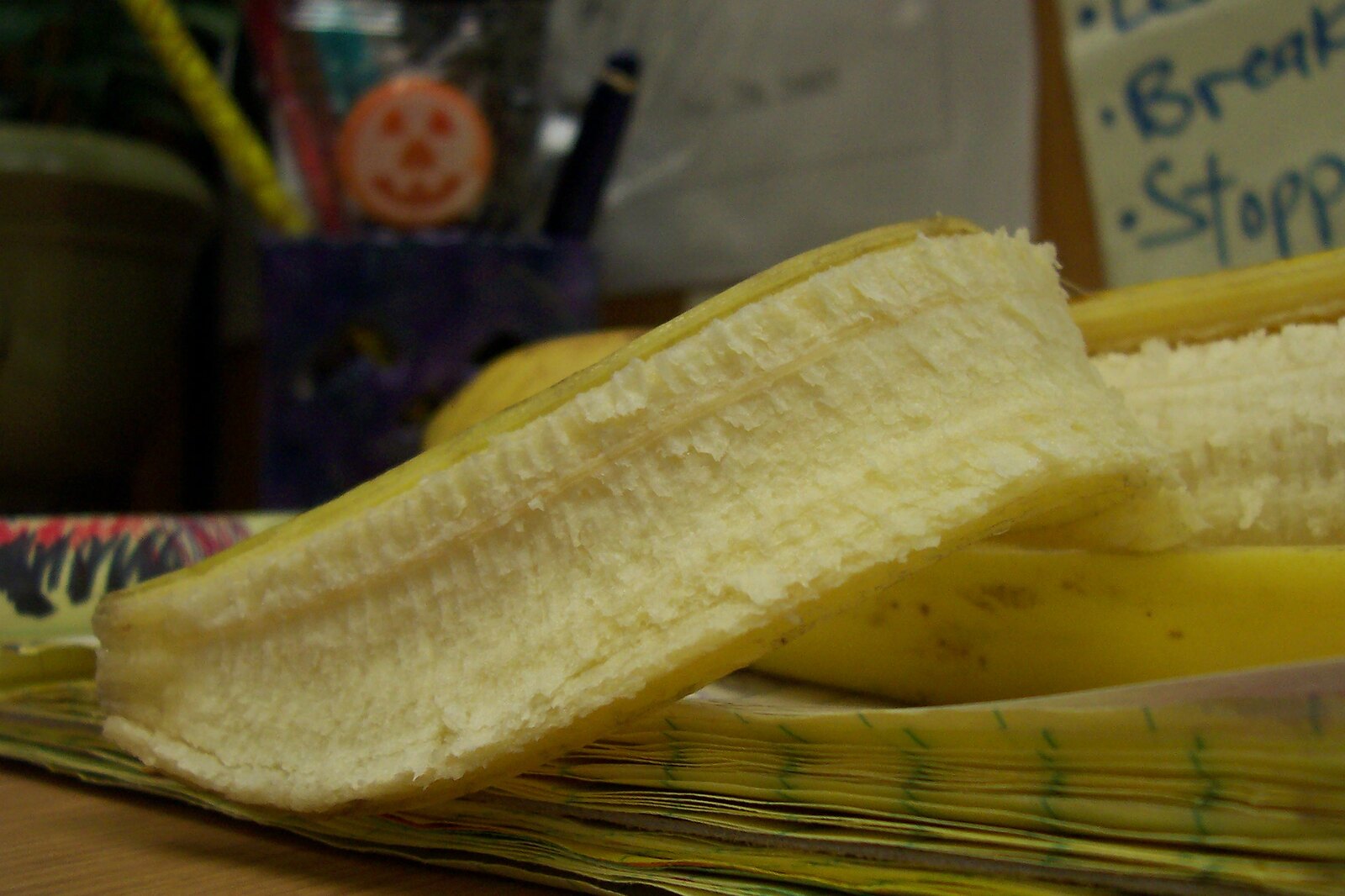The photograph showcases a partially peeled banana, with about a quarter or a fifth of the peel pulled back, revealing the fruit still encased within. The banana is resting on top of a ruled notepad, creating a casual yet organized workspace scene. Directly behind the notepad is a pencil holder, brimming with various pencils and pens, adding a sense of busy productivity. Among the pens and pencils is a conspicuous jack-o-lantern, possibly a decorative oversized sucker or novelty item, lending a playful touch. In the background, papers are pinned up on what appears to be a cork board, some secured with pens. The pinned papers feature legible text, including the words "BREAK" and part of a longer word starting with "STOP," where only the first two letters and the last “P” are clearly visible. The overall setup suggests a working or study environment with a hint of whimsy and seasonal decoration.